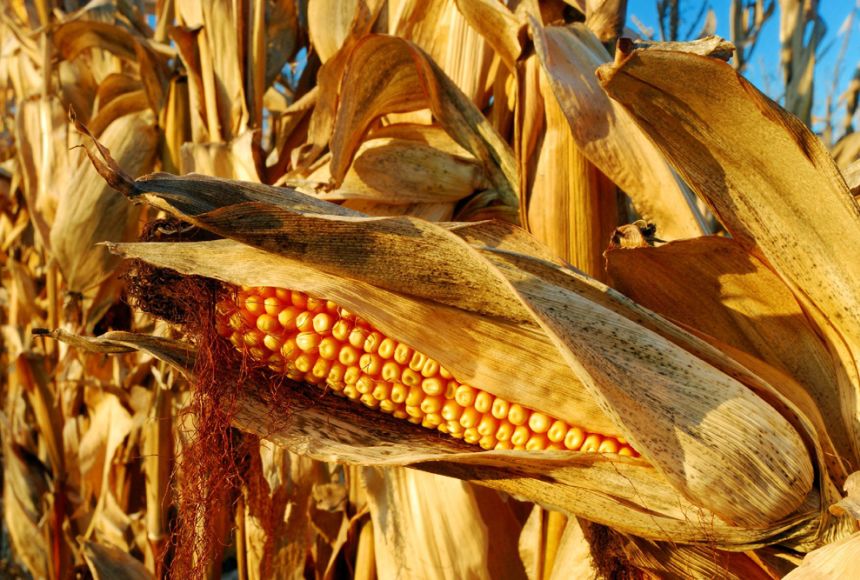The photograph captures a detailed, close-up view of an ear of corn in a field, emphasizing the vibrant yet weathered nature of the produce. The corn's husk is yellow and dried, partially peeled back to reveal the cob, which glows with an orangish-yellow hue reminiscent of pearls in the sunlight. The corn's silk strands are strikingly red, adding a pop of color to the earthy scene. The background showcases more dried, yellow-brown husks and hints of blue sky in the upper right corner, suggesting a clear day. The landscape orientation and macro focus draw the viewer's attention to the texture of the kernels, some of which appear slightly sunken and darker, indicating both the late season and potential drought conditions. The overall scene evokes a sense of autumn harvest, highlighting the cycles of growth and decline in the agricultural setting.